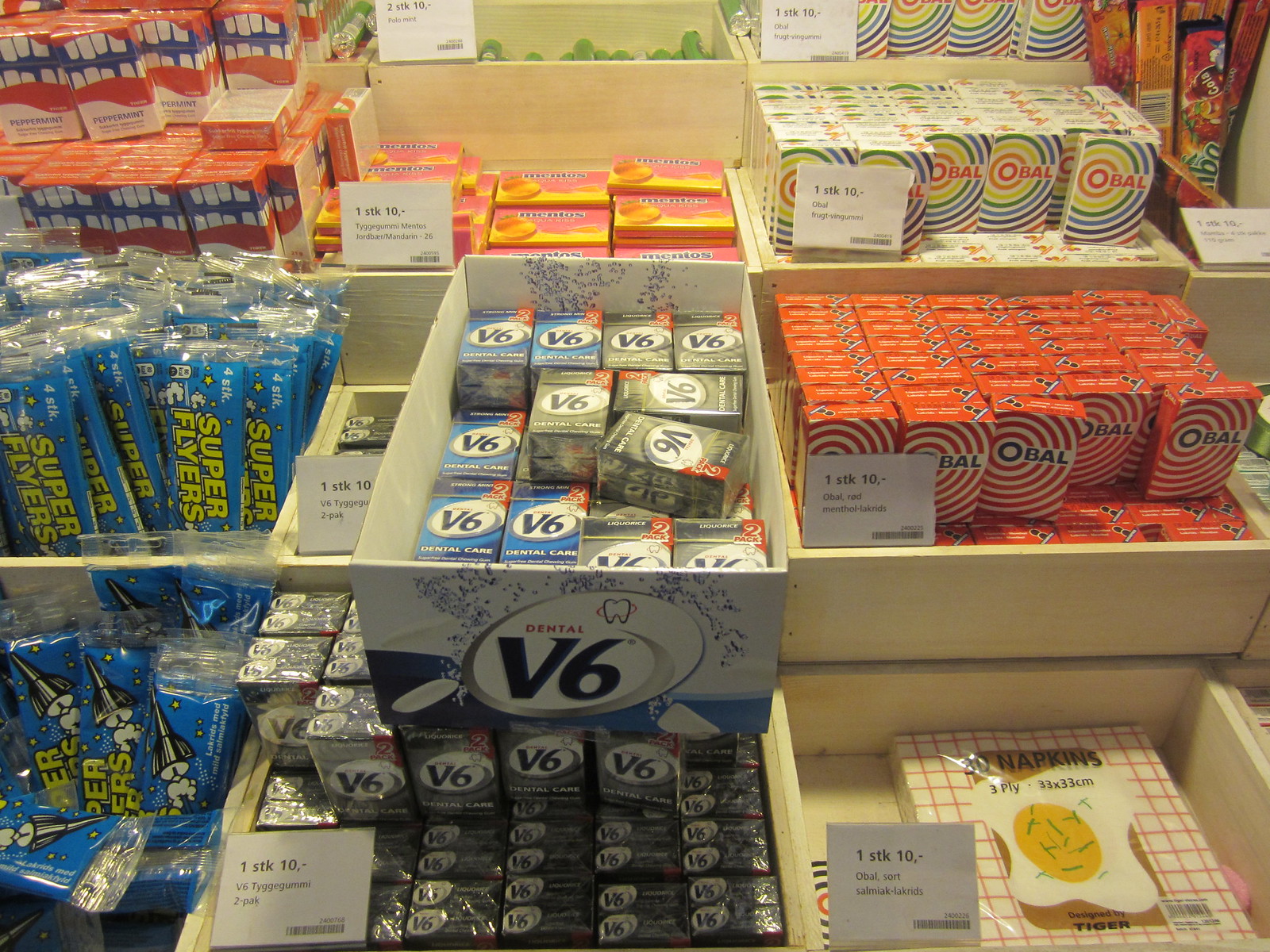In the image, a variety of small products are meticulously displayed as if in a retail store. The items are organized into six distinct sections, each filled with products of the same brand or type, stacked neatly in wooden boxes. At the center of the display is a box labeled "Dental V6," likely a dental product, with its packaging featuring a picture of a tooth. On the left, there is a box of products called "Super Flyers," contained in blue packaging, while to the right, labeled "Obal," is another set presented in a distinctive orange box with an orange and white target circle, and further behind that, a similar design but in rainbow colors. A stack of napkins for sale occupies the front right side. Each product section has small signs propped up in front displaying the price, with text like "1STK10" prominently visible. The colors of the products range from red, white, blue, gray, light blue, yellow, and a tannish white, all arranged closely together to create an inviting and orderly display.